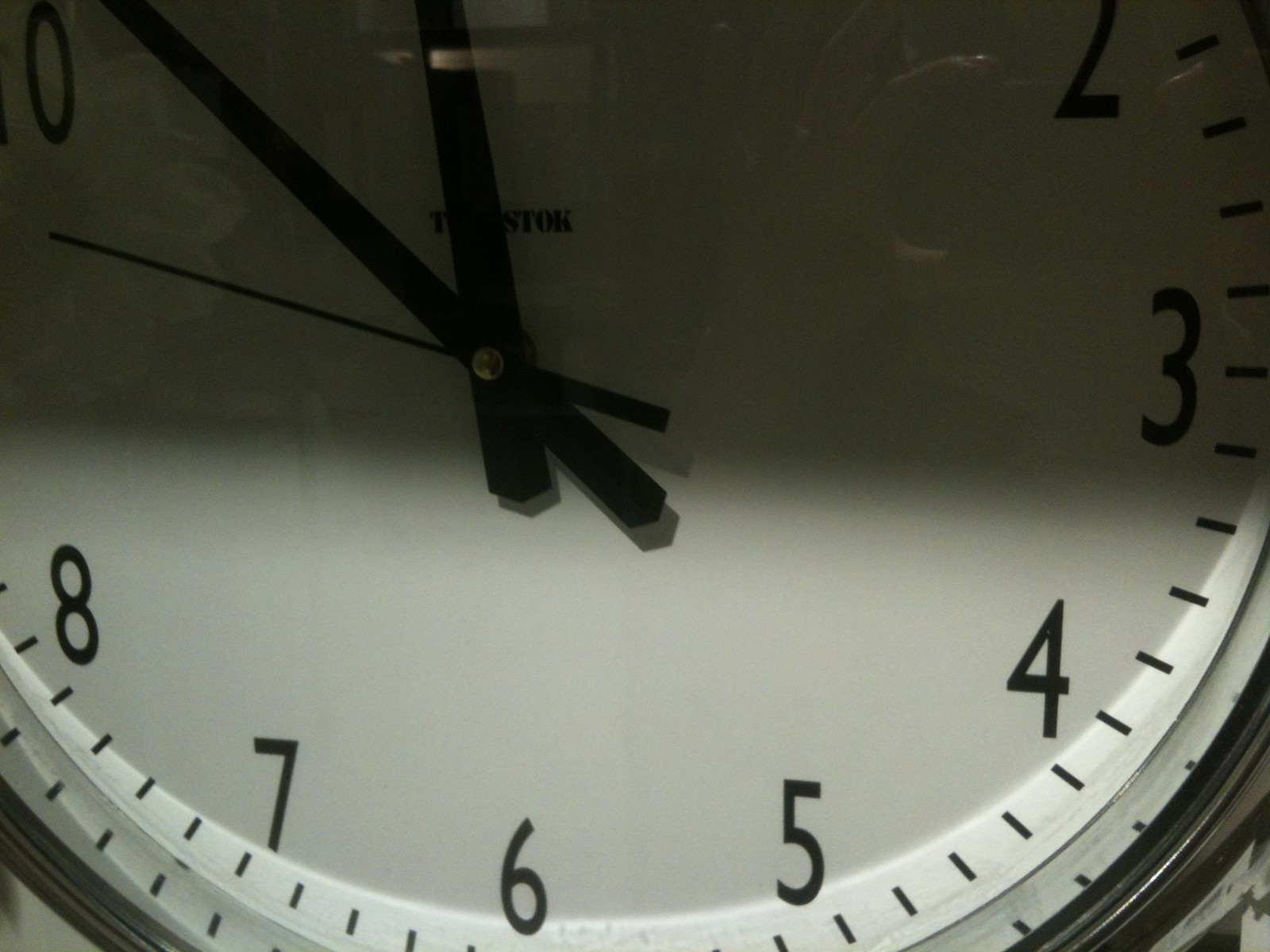The photograph captures the middle to lower portion of an analog clock, featuring a white face adorned with distinct black numerals. The clock is demarcated with precise minute markers that encircle the rim. The slender, black hour and minute hands extend gracefully, complemented by an exceptionally thin, needle-like black second hand. The outer face of the clock is either clear glass or plastic, noted for its high reflectivity, capturing light and the minute markers in its reflection. The clock's edge is trimmed in chrome, adding a touch of elegance. Partially obscured by one of the hands is a brand name engraved on the clock face, starting with the letter 'T' and ending with the letters 'STOK.'